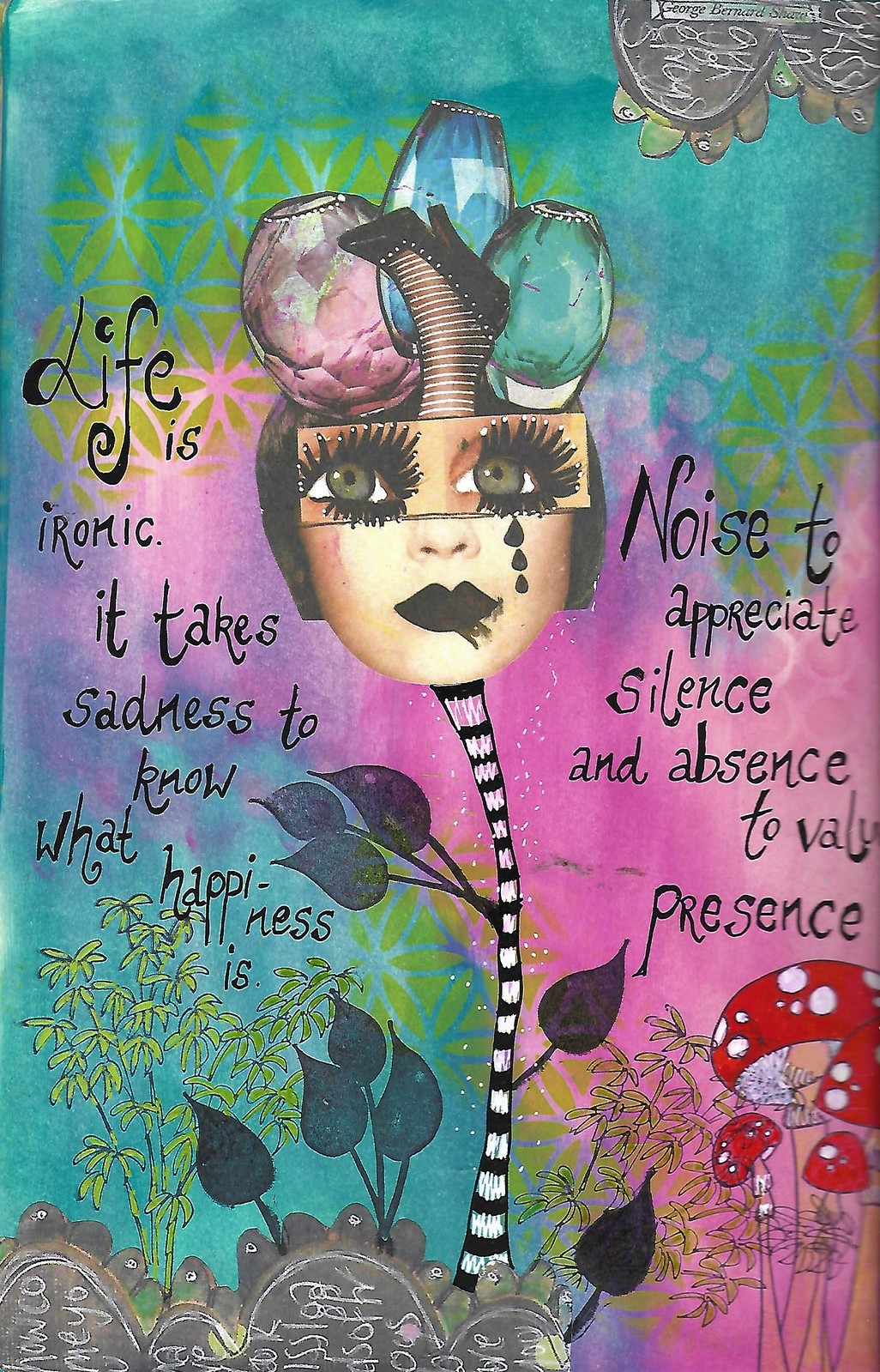This is an abstract and modern artwork featuring a woman's face superimposed over a floral motif. The central figure, a woman's face, is characterized by distinctive black lipstick, dramatic black eyelashes, and tears of black streaming down from her eyes. An unusual element of the piece is an upside-down foot clad in a high heel, protruding from the top of her head, accompanied by some ambiguous glass candle holder-like objects. The background is a vibrant collage of colors, incorporating shades of green, violet, yellow, blue, pink, and brown. In the bottom right corner, a cluster of red mushrooms with white spots can be seen, along with leaves extending from the flower. Two textual elements frame the central image: on the left, in fancy cursive black font, "Life is ironic. It takes sadness to know what happiness is," and on the right, "Noise to appreciate silence and absence to value presence." The artwork as a whole conveys a surreal and thought-provoking visual narrative.